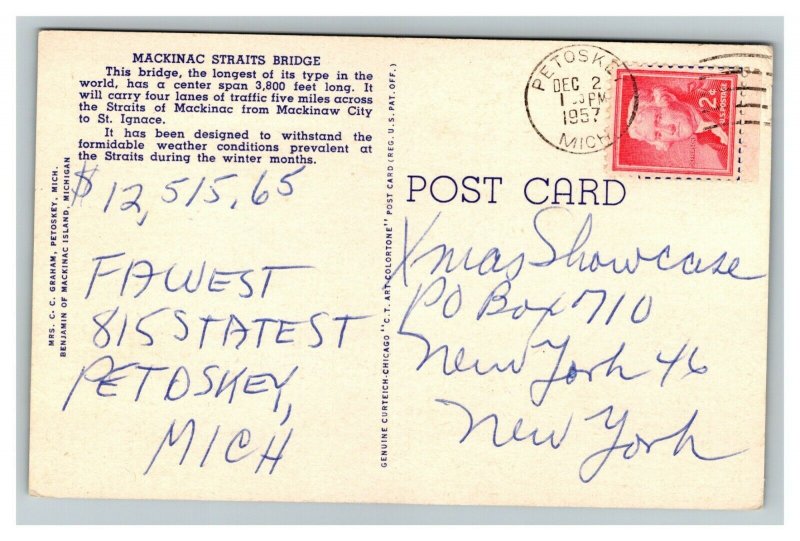The image depicts the back of an old postcard, possibly pink in color, lying on a gray surface. The postcard features numerous details, both printed and handwritten. At the top left corner, in blue capital letters, it says "MACKINAC STRAITS BRIDGE." Below that, it includes two paragraphs in purple text describing the bridge: "This bridge, the longest of its type in the world, has a center span 3,800 feet long. It will carry four lanes of traffic five miles across the Straits of Mackinac from Mackinac City to St. Ignace. It has been designed to withstand the formidable weather conditions prevalent at the Straits during the winter months."

Further down on the left side, handwritten in blue ink, it says "$12,515.65" and gives an address: "Far West 815 State Street, Petoskey, Michigan." The center of the postcard divides the left and right halves with a line of purple print that’s difficult to read.

On the right side, in the top corner, there is a red two-cent U.S. postage stamp featuring a man, possibly Jefferson, with white hair and dark clothing. The stamp is canceled by a black postmark that reads "Petoskey, December 2, 1957, MICH." Beneath the stamp, in large blue letters, it says "POSTCARD." Below that, handwritten, is an address: "XMAS Showcase, P.O. Box 710, New York, 46, New York."

The backdrop of the postcard appears to be light blue, further highlighting its age and wear.